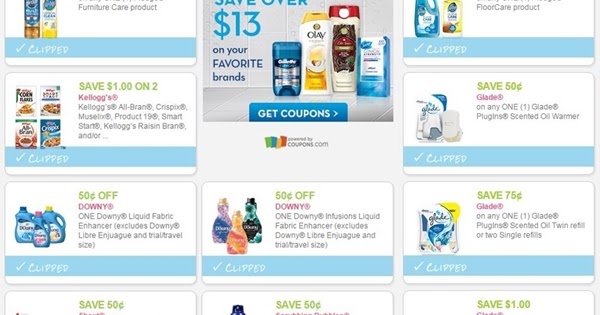This image depicts a webpage featuring a collection of coupons organized in a grid layout. The majority of the background of each coupon is white, while the main body of the page is a pale gray. Each coupon is demarcated with a light blue bar at the bottom, displaying savings amounts in light green text. The product names are highlighted in pink, and additional information is presented in black.

The layout consists of three columns with two full rows and three partial rows of coupons. On the left-hand side of the first row, there is a partially visible product. Below it, there is a coupon for Kellogg's offering a $1 saving on the purchase of two items, with a note indicating that this coupon has been clipped. The next coupon below offers $0.50 off Downy products, which has also been clipped. Following this is another $0.50 savings coupon, though the product is not visible.

In the middle column, at the top, there is a large promotional banner inviting users to "Get Coupons" and "Save up to $13 on your favorite brands," accompanied by a small logo. Below this banner are two Downy coupons: one offering a 50% discount and another top coupon.

On the far right-hand side of the first row, a coupon for a floor cleaning product is visible. In the second row, there is a coupon offering $0.50 off Glade products, and at the bottom right-hand corner of the page, another Glade coupon provides a $0.75 discount. Additionally, partially visible at the bottom in the right corner is a coupon offering a $1 saving.